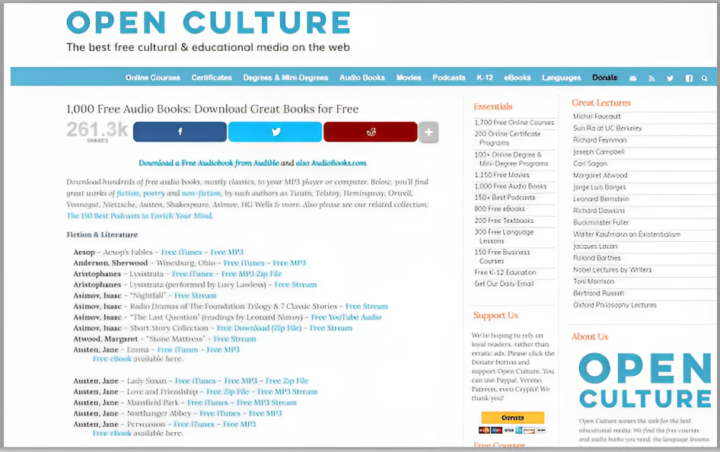This screenshot captures the homepage of Open Culture, a renowned platform offering an extensive collection of free cultural and educational media. Dominating the center of the page is a headline that emphasizes the availability of 1,000 free audiobooks for download, catering to avid readers. The top navigation bar features various clickable icons, facilitating easy access to categories such as certificates, degrees, mini-degrees, and audiobooks. The site appears to operate as a nonprofit, as highlighted by the donation prompts strategically placed around the interface, including options for credit card contributions.

Central to the page is a section showcasing the sheer volume of content available, noting over 261,000 downloads to date. The literary collection starts alphabetically with titles like "Aesop's Fables" and continues through works by Sherwood Anderson and Jane Austen, allowing users to download these classic texts directly. To the right, additional features are displayed, including free movies and language lessons, underscoring the site's diverse offerings. The homepage of Open Culture solidifies its reputation as a vital resource for free educational and cultural materials while encouraging user donations to sustain its operations.